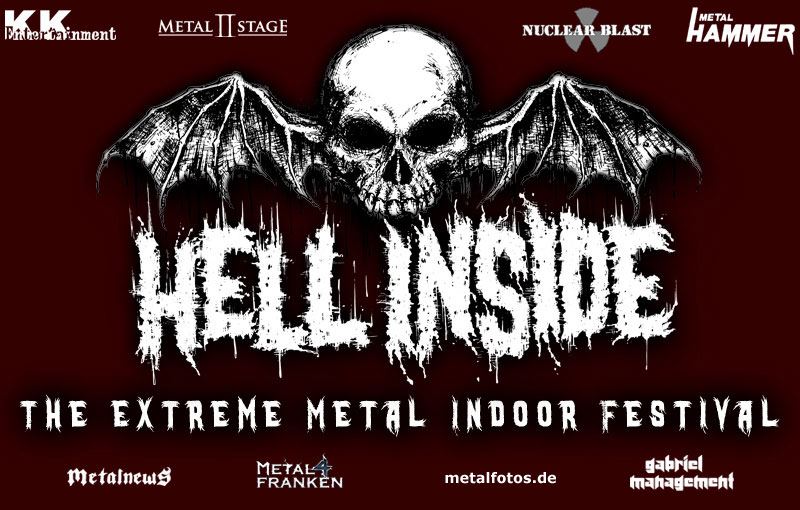This is a poster for a heavy metal music festival, rectangular in shape, featuring a striking dark blood-red maroon background. Dominating the center is a black and white illustration of a human skull adorned with bat wings extending from either side. Directly beneath this graphic, in large, white, scratchy capital letters, is the title "HELL INSIDE." Below this title, the text announces "THE EXTREME METAL INDOOR FESTIVAL," also in white. The top of the poster showcases an array of logos in white, belonging to KK Entertainment, Metal 2 Stage, Nuclear Blast (with a radioactive symbol), and Metal Hammer. Additional logos and band names are displayed below the festival title, including Metal News, Metal Franken, MetalPhotos.de, and Gabriel Management, all contributing to the festival's dark and intense aesthetic.